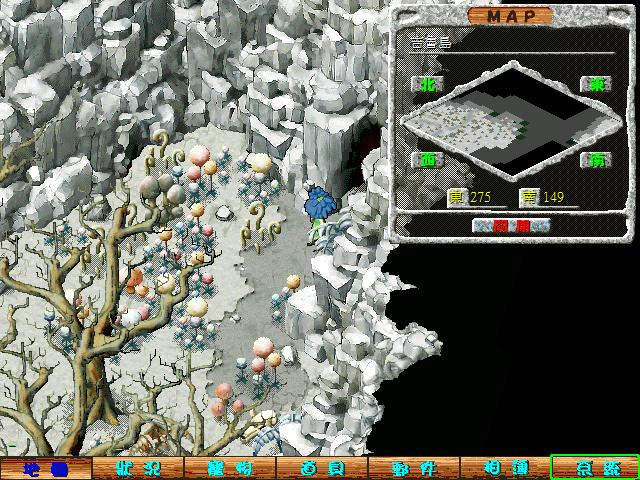This detailed still shot from a video game depicts a rocky landscape dominated by stone formations and a gully filled with various plants. In the left-hand section, there's a thick-trunked, leafless tree with branches that extend outward, surrounded by an array of colorful orbs mounted on poles in pink, blue, and yellow. The ground transitions from a very pale green on the left to a pale gray on the right.

A significant feature is a cave entrance located amid the stone formations, where a character with blue hair, resembling a flower, is seen entering. Near this entrance, peculiar plants resembling cacti and blue-gray foliage with orb-like growths add to the surreal environment. Yellow and orange shrubs are also visible in this area.

In the upper right-hand corner of the screenshot, a black panel contains a gray square, outlined in stone and topped with wood. This square functions as an in-game map. "Map" is written in dark brown text at the top, accompanied by white Asian characters and various symbols. The map includes gray rectangles with green centers and a white diamond shape featuring black and gray patches. Numbers 275 and 149 are positioned at the bottom of this panel.

The bottom part of the image features a wooden border adorned with Asian writing. Additional symbols appear in dark blue and sky blue, with a green-lined symbol at the lower right corner, enhancing the intricacy and immersive feel of the game interface.